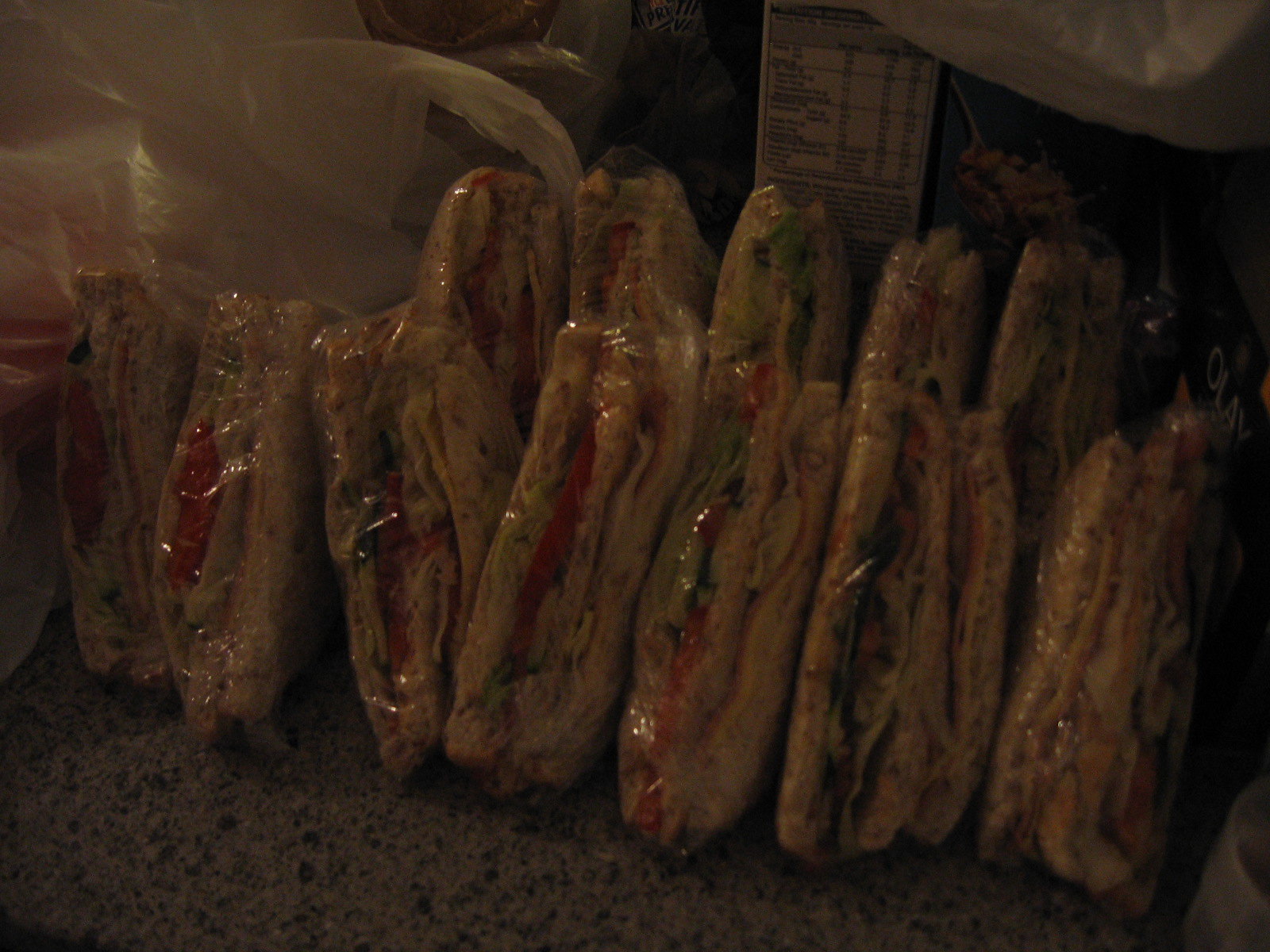A very dark and slightly grainy color photograph depicts twelve triangular sandwiches meticulously stacked in two diagonal rows. Each sandwich, wrapped tightly in plastic wrap or clear cellophane, showcases visible layers of sliced bread, iceberg lettuce, tomato, deli meat, and possibly cheese. The crusts have been removed, presenting neatly cut edges. The sandwiches rest on a mottled gray countertop or table, with light reflecting off the plastic. Toward the back left corner, a grocery-style plastic bag is faintly visible. The upper part of the image plunges into darkness, obscuring any background details.